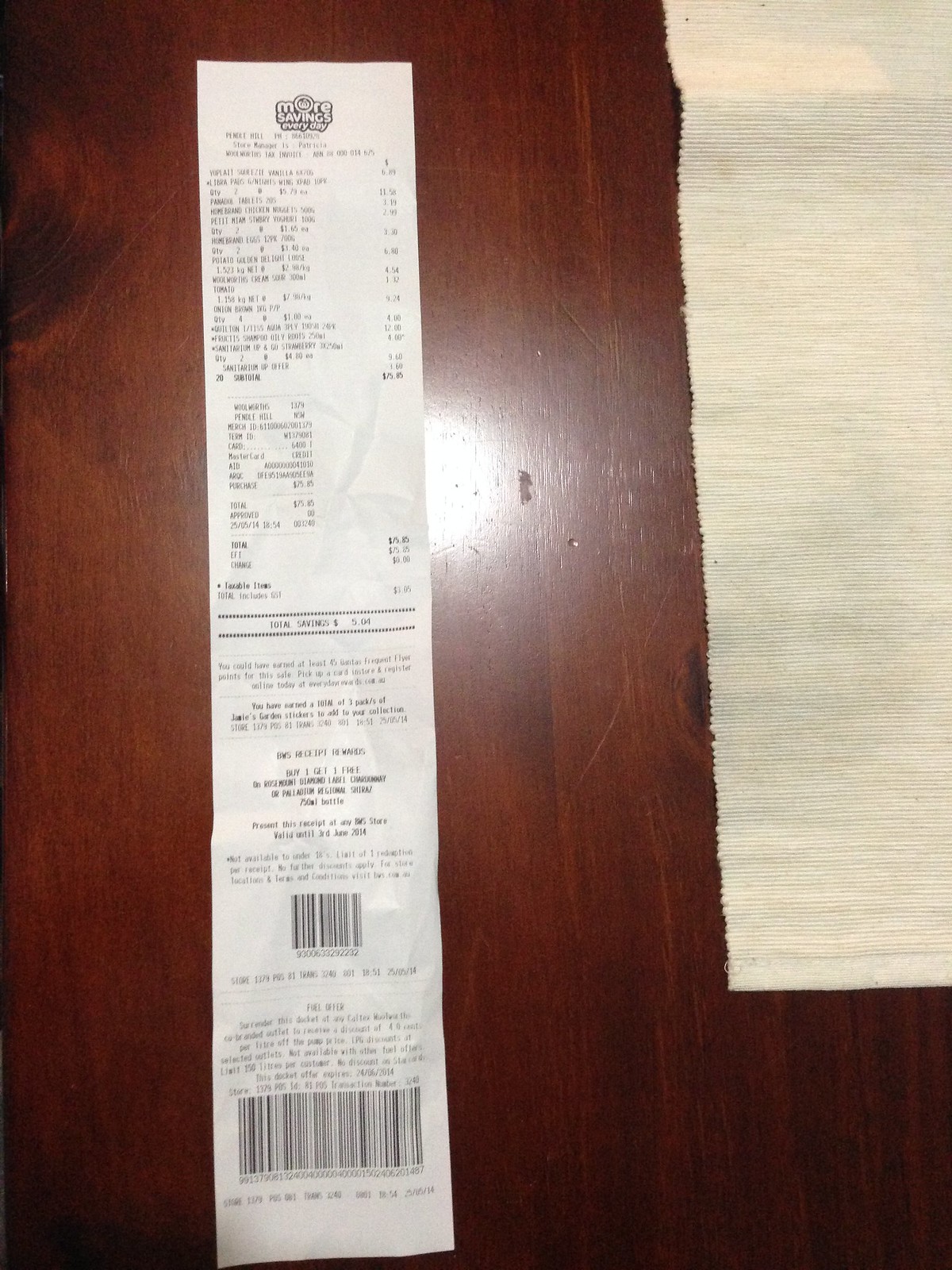This image features a long, white receipt placed on a brown wooden table. The table has an off-white table runner, but the receipt is positioned directly on the exposed wood. The photograph is slightly blurry, making the text difficult to read. However, the top of the receipt is visible and includes the phrase "more savings every day" followed by a list of purchased items and their prices. Midway down the receipt, the phrase "total savings 501" is identifiable. The receipt also contains two black UPC codes, one situated at the bottom and the other further up, possibly indicating sections for returns or gift receipts.